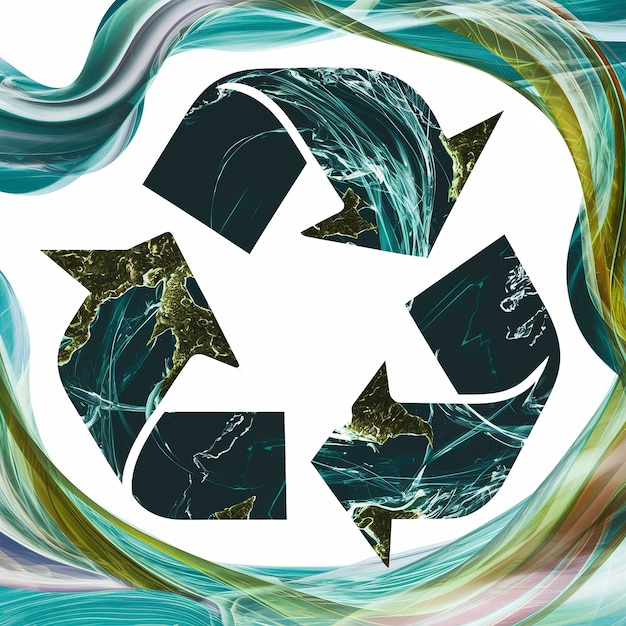The image features a square graphic showcasing the iconic recycling symbol centered on a white background. The recycling symbol is composed of three curved arrows forming a triangular shape, each arrow appearing to point towards the center in a clockwise direction. The arrows themselves are adorned with intricate artwork resembling a map, with dark blue and green hues interspersed with white swirls, adding a textured, geographic feel to the design. Surrounding the white background is a vibrant border composed of swirling, tendril-like patterns, mimicking the fluid motion of water. These decorative edges boast a rich palette of green, blue, purple, orange, red, pink, teal, and yellow colors, creating an artistic frame that enhances the central recycling motif.